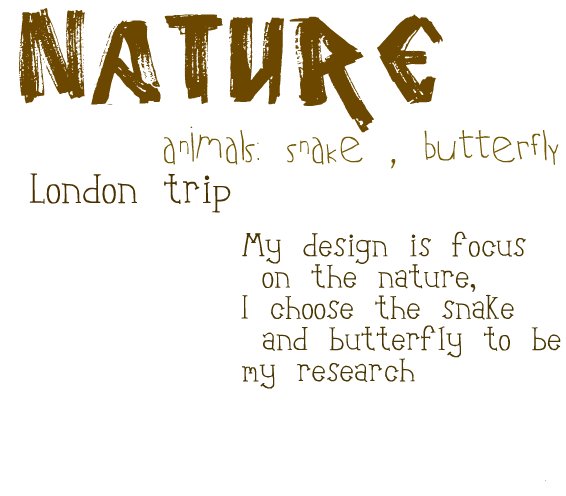The image features a minimalist design with a stark white background and brown text. At the top, the word "nature" is prominently displayed in large, bold letters that mimic brush strokes, featuring visible streaks for an artistic effect, though it appears to be computer-generated. Beneath "nature," the text "ANIMALS: SNAKE, BUTTERFLY" is written in a cursive-like, uneven font, giving the impression of being hand-written. Further down, the words "LONDON TRIP" appear in a standard printed format. The final line reads, "MY DESIGN IS FOCUSED ON THE NATURE. I CHOOSE THE SNAKE AND BUTTERFLY TO BE MY RESEARCH," conveying the theme and intent of the design. The overall layout is orderly, yet the varying fonts add a touch of creative diversity.